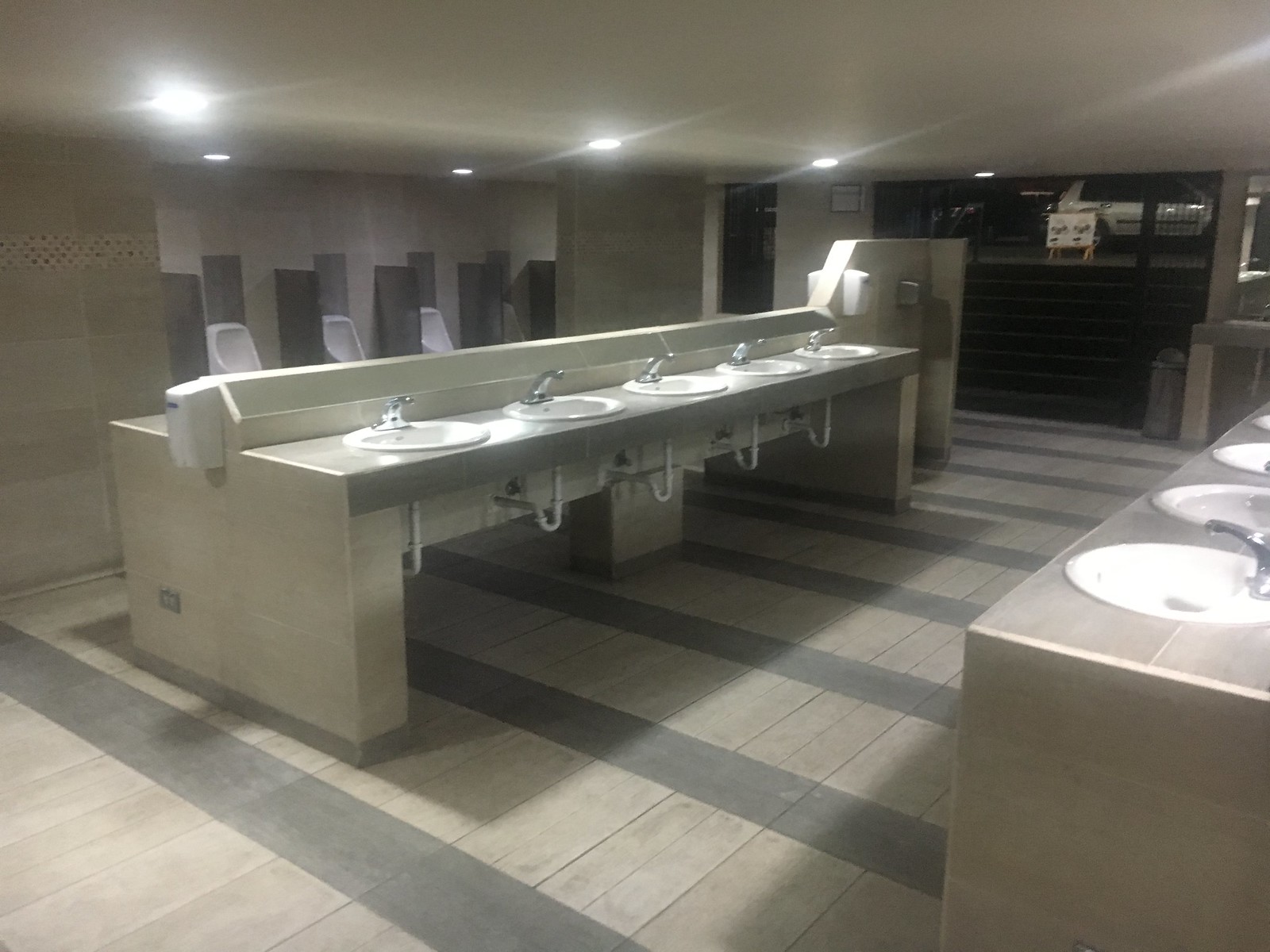A photograph of a slightly dark and deserted men's public restroom. The floor features wide and narrow gray stripes set in a diagonal pattern from the bottom left to the top right. At the top right corner of the room, steps lead up and out to what appears to be a city street, with a car visible at the exit. The ceiling is gray, dotted with six scattered recessed lights.

In the center of the image, there is a dual-sided station with five white sinks, each fitted with a silver tap and exposed white plumbing beneath the silver countertop. On the left end of this central sink station, there's a soap dispenser and possibly a paper towel dispenser. To the left, along the wall, there are three white urinals with dark-colored partitions above them. In the bottom right corner of the image, additional sinks are visible—one fully and two partially—all white with silver faucets. The walls are gray tiles with slight decorative edges. The photograph captures a utilitarian, minimally decorated restroom, with practical fixtures and a muted color scheme, illuminated by multiple can lights.